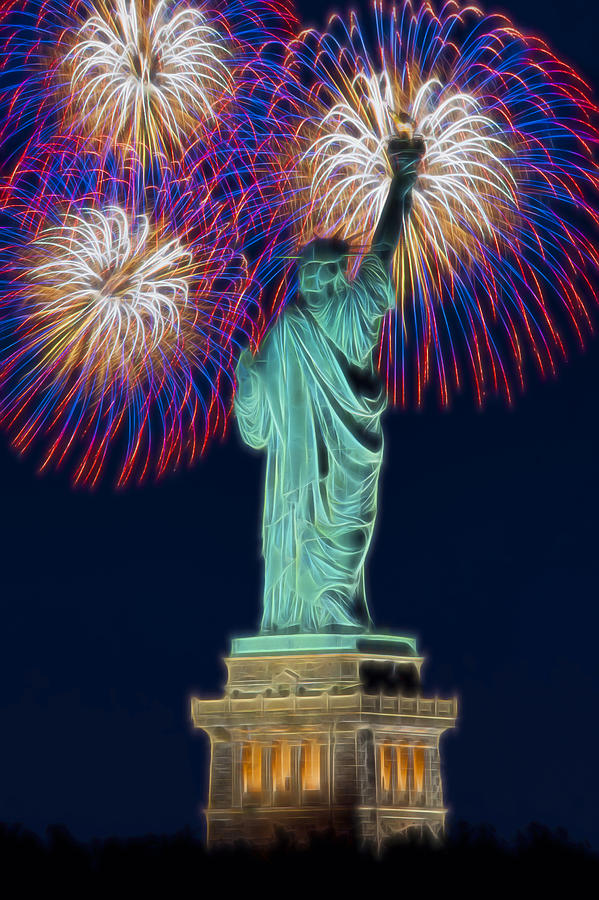This striking image depicts the Statue of Liberty at nighttime, illuminated against a black sky and showcasing a vivid fireworks display. The statue, rendered in a bright green hue, stands on a brown-lit platform with windows glowing orange. Its back is facing us, with the famous torch held high. Above the statue's head, beams of light radiate like a crown, adding a majestic touch to the scene. The fireworks explode in a dazzling array of colors—red, white, blue, yellow, and purple—creating a celebratory tribute likely to the 4th of July. The lower half of the image is dominated by the solid black of the night, contrasting with the vibrant explosions and lending a dramatic effect to this digital or artistic rendition. The composition captures both the serene grandeur of Lady Liberty and the dynamic beauty of the fireworks, making it a visually captivating tribute to the iconic monument.